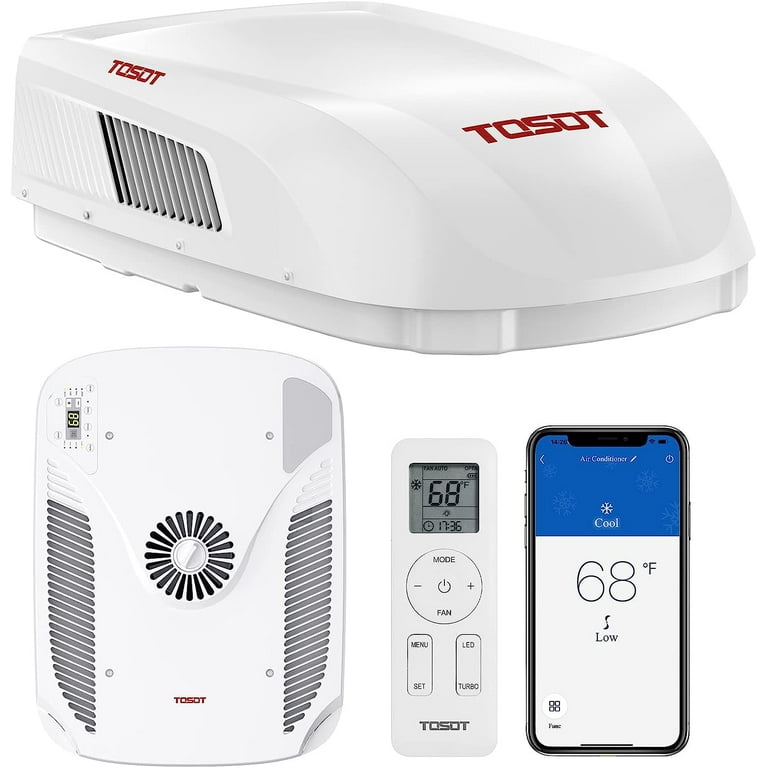This image showcases a detailed view of an air conditioner, specifically designed for RVs, branded TOSOT in bold red letters on a sleek white shell. The topmost and largest section of the photo highlights the aerodynamic pod-shaped structure with vents on the sides. The subsequent images provide various perspectives: one reveals the underside featuring a sun-shaped vent, diagonal vents, and a remote control labeled with "mode" and "fan." Another image displays a thermostat reading 68 degrees Fahrenheit. Additionally, a smartphone interface depicting the same temperature setting indicates that the device can be controlled via a mobile app. This comprehensive depiction emphasizes the unit's design, functionality, and modern connectivity options.